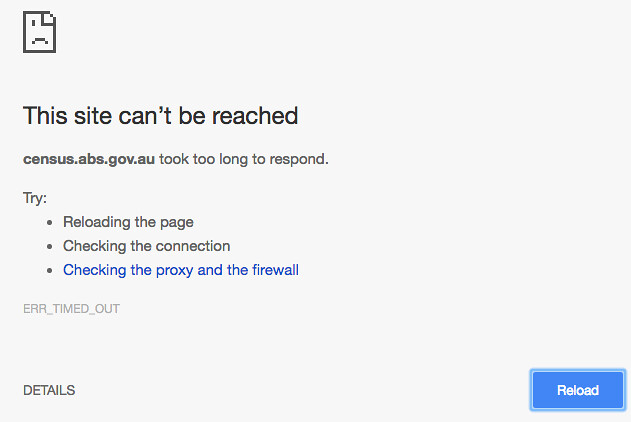This image depicts a screenshot of an error message on a computer or mobile device. The background is light gray. In the top left corner, there's a low-resolution icon of a piece of paper with a top-right folded corner, featuring an anthropomorphized face with one eye in the top left and a frown at the bottom. 

Below this icon, the largest text reads, "This site can't be reached." Following this, in smaller text, is the message, "census.abs.gov.au took too long to respond." Beneath this, the word "Try" precedes three bullet points; the first two in gray text suggesting "Reloading the page" and "Checking the connection," and the third in blue text recommending "Checking the proxy and the firewall." 

Further below, in light gray text, is the error code "ERR_TIMED_OUT." In the bottom left corner, "Details" is written in dark gray text. On the bottom right, a blue button is present. This button has a medium blue fill, a thin white outline, and a translucent blue gradient resembling a shadow or aura surrounding it. Centered within the button, the word "Reload," written in capitalized white text, invites the user to retry loading the page.

The image's layout features significant negative space above and to the right of the text, maintaining a clean and minimalistic appearance.